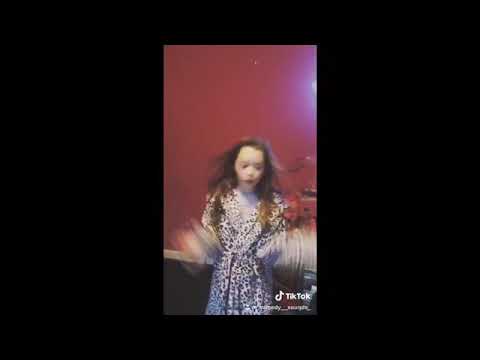A screenshot from a TikTok video featuring a young girl with white skin and long, dark brown hair flowing down to her chest. She is wearing a mostly white bathrobe with black speckles, resembling a cheetah print. The image is centered with a large black border and shows the TikTok logo along with the 'TikTok' label in the bottom right corner. The girl's face and hands are blurred due to her rapid movements, creating a sense of motion. She stands on a dark-colored floor with a white trim, in front of a maroon-colored wall. In the upper right corner, there's a blue glowing object that casts a faint blue shadow on the wall.